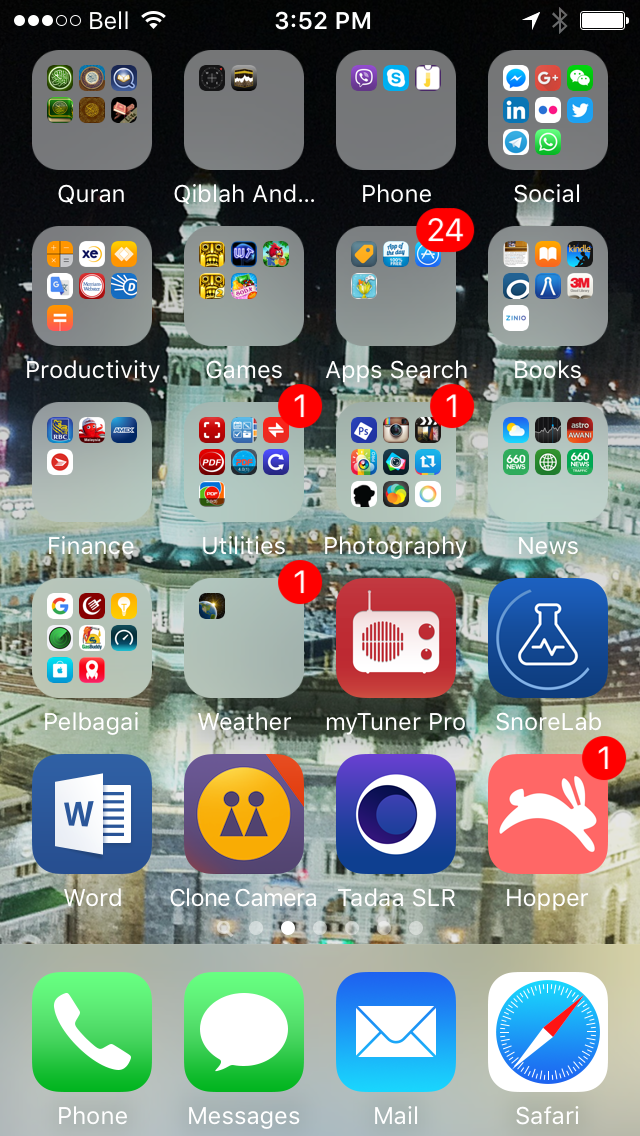This image is a screenshot of an iPhone screen, identified by the presence of the Safari app in the bottom right corner. The status bar at the top displays the service provider "Bell," a centered time reading "3:52 PM," and the battery indicator in the top right. 

The background image appears to be a night-time photograph of Mecca, characterized by prominent buildings and a predominantly black upper section. The apps are organized into categorized folders: 

- **Top Left Folder**: Related to the Quran, hinting at the relevance of the background image.
- **Other Folders**: Including categories such as Phone, Social, Productivity, Games, App Search, Books, Finance, Utilities, Photography, and News.
- **Individual Apps**: MyTuner Pro (radio app), Snorlab (sleep tracking), Word, Clone Camera, an SLR camera app, and Hopper (travel deals).

Additionally, common iPhone apps like Phone, Messages, Mail, and Safari are also visible, giving a comprehensive view of the phone's organized and varied app usage.